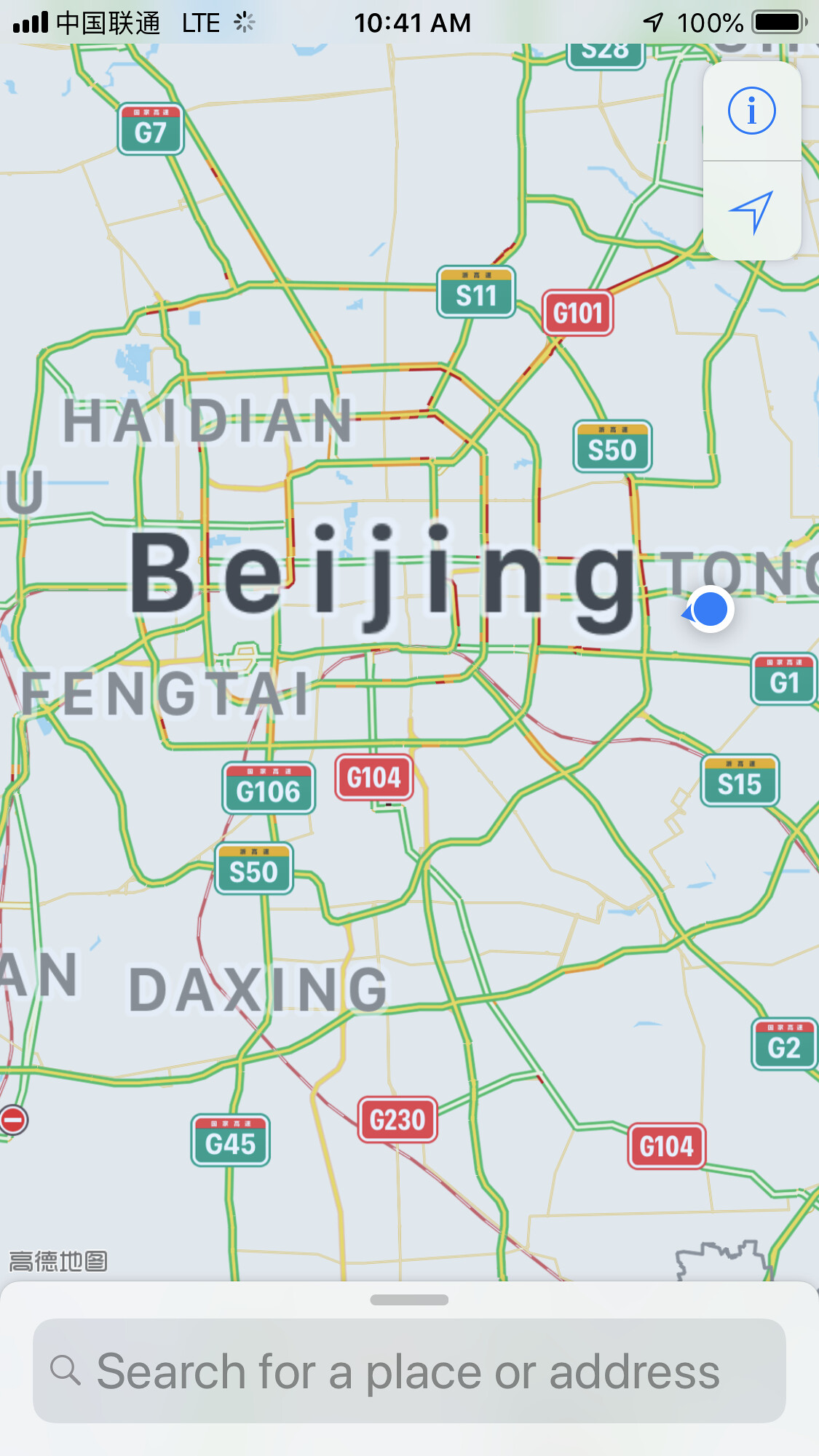The image showcases the screen of a portable device, likely a cell phone, smartphone, or tablet, as indicated by the icons on the top edge. These icons include signal strength bars, "LTE" connectivity, the current time of 10:41 AM, and a battery power indicator showing 100%. The screen displays a detailed map of Beijing, China, highlighting various urban and suburban regions. Prominently labeled areas include Haidian, Fengtai, and Daxing. 

The map details an intricate network of highways, with some routes marked in green and others in red, indicating different traffic conditions or road statuses. A significant feature is the loop highway labeled S50, which transitions into S11. Major roads extending from the loop include highways G101 and G104, among others. Additionally, multiple loops and crossroads are highlighted within the city's layout, providing a comprehensive overview of Beijing's major transportation routes.